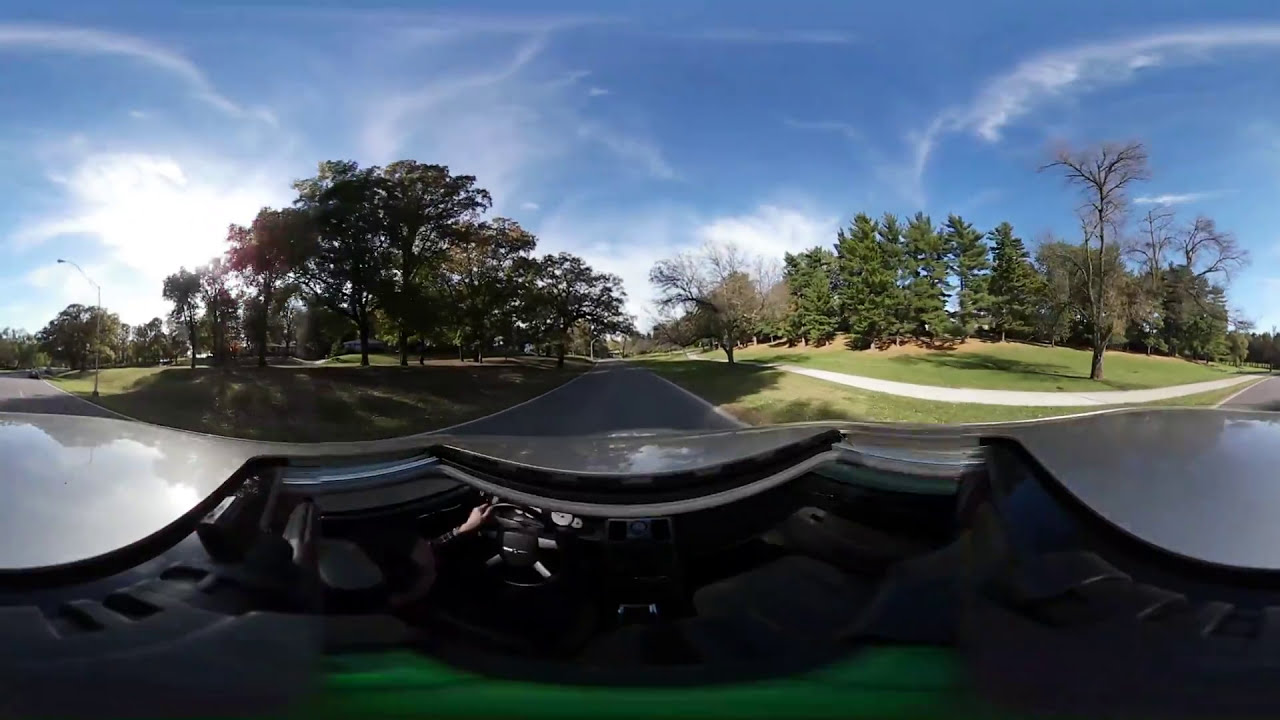This image captured from inside an automobile appears to have been taken using 360 imaging, providing a wide and somewhat warped view from the driver’s perspective. The lower portion of the photo reveals the dark gray exterior of the car, the steering wheel, and a person’s hand on the left side. As the view extends outward, you see a two-lane road with no center divide lines threading through a lush, green area that resembles a golf course or a park, flanked by grassy areas and numerous trees on both sides. The road seen from the car continues straight before curving to the left near the top of the photo. An intersecting main road, marked with yellow lines and equipped with streetlights, appears further ahead. Sporadic clouds dot the exceptionally light blue sky, amplifying the serene ambiance of this verdant corridor. The image captures not just the scenic greenery but also the dynamic, immersive quality typical of 360-degree photography, giving the viewer a panoramic experience of the landscape.